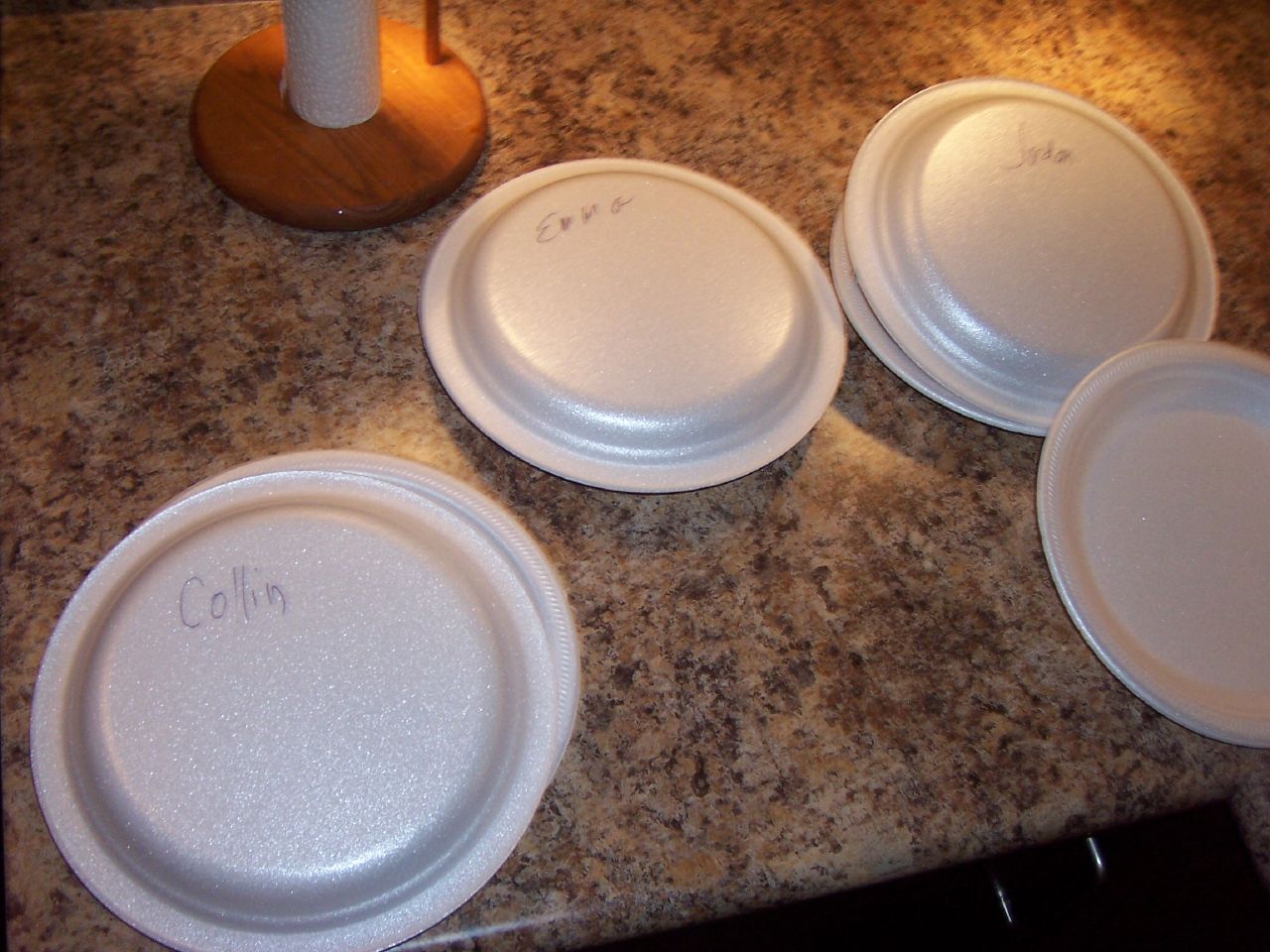The image depicts a granite countertop with a mix of gray, brown, and black hues. Prominently placed on the counter are four sets of Styrofoam plates. Each set comprises two plates: a lower one holding food and an upside-down plate on top acting as a cover. The plates are labeled with names written in marker. From left to right, the labels visible are "Colin," "Emma," and "Judah." The fourth plate set, positioned on the lower right, consists of just a single, uncovered plate facing up. Additionally, a wooden paper towel holder with a partially used roll of textured paper towels is partially visible in the upper left corner of the image.